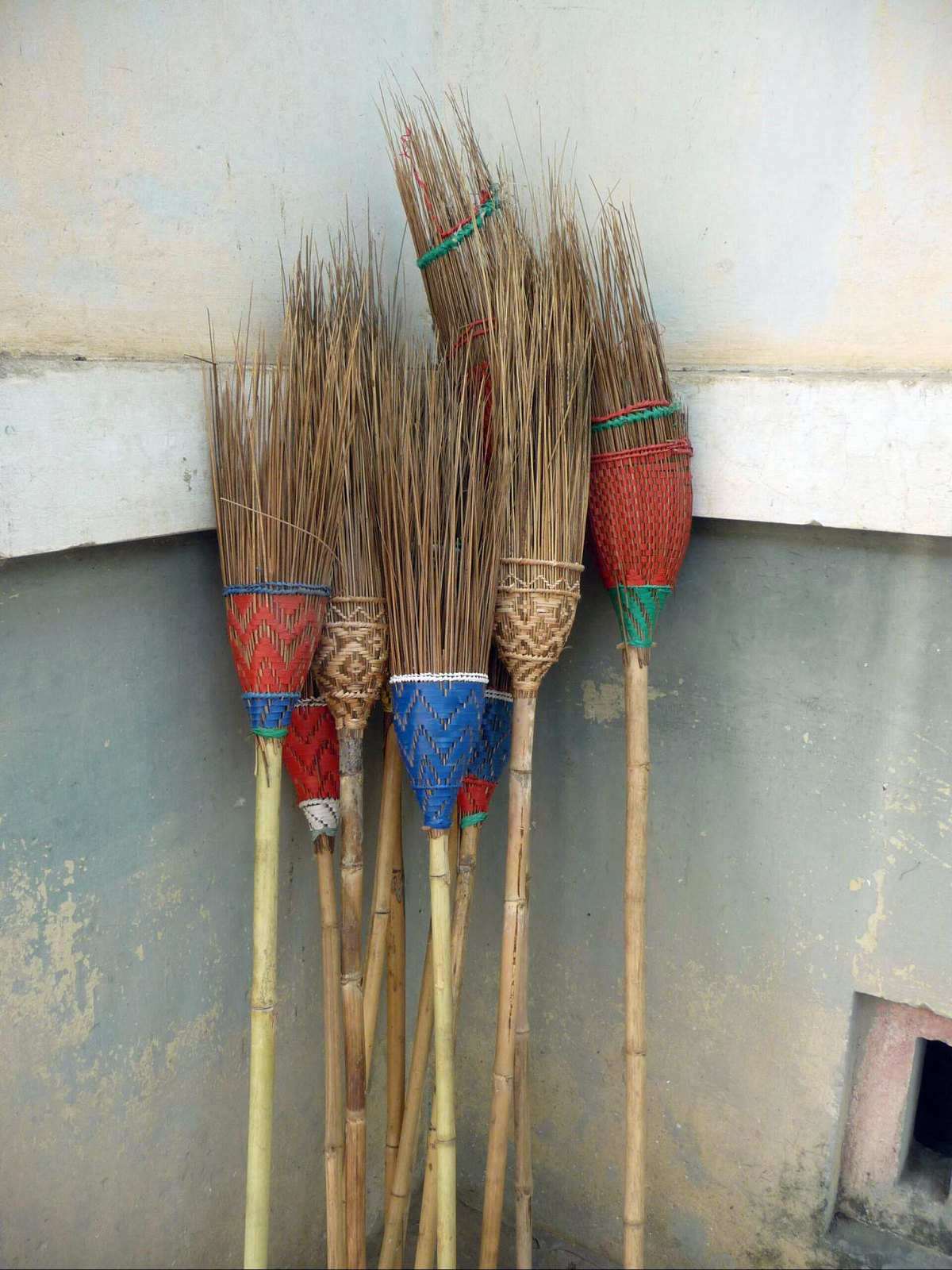This photograph captures a group of traditional handmade brooms, likely from Asia, showcased in a vivid and detailed manner. Each broom features a bamboo handle and a sweeping section composed of sticks or branches, bound together with colorful yarn or string. The bindings, which come in hues of red, blue, green, and natural straw color, secure the sweepers to the handles at various points, creating an intricate and colorful pattern. These brooms, numbering seven or eight, are leaning against the corner of a building, specifically against a wall with a visibly weathered gray and bluish-gray facade. The top half of the wall is white, though aged and stained, indicating an outdoor setting. A small square opening is partially visible on the bottom right portion of the photograph. The entire scene emphasizes the rustic, handcrafted nature of the brooms against the backdrop of the faded, peeling paint on the building.